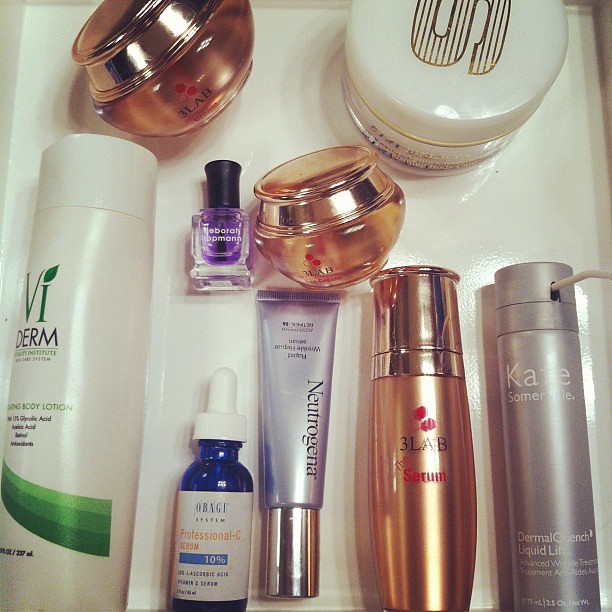A meticulously arranged display of various cosmetics sits on a white tabletop. The assortment includes both small and large containers, each serving a unique purpose in skincare. At the forefront, a white tube adorned with green streaks is labeled 'Viderm.' Beside it, a small blue glass bottle with a precision dropper, identified as 'Professional-C Serum,' suggests a high-quality facial serum. A small tube of Neutrogena, purpose unspecified but possibly for the face or hair, lies nearby. Adding a touch of luxury, a gold bottle with red accents and bold black lettering reads '3Lab.' Adjacent to this is a product branded 'Kate,' spelled out in bold letters, likely a liquid dermal treatment. Behind these items, a bottle resembling a nail polish container holds a striking purple liquid. The ensemble is rounded off with three jars—two small, one larger—all likely containing various facial creams or treatments. This assortment reflects a comprehensive approach to skincare, featuring a mix of high-end and everyday beauty solutions.